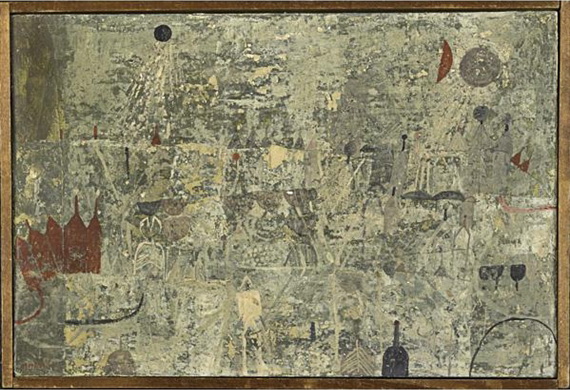The painting is an abstract composition featuring a blend of light gray, dark gray, and brown hues, with occasional splashes of yellow and light green. Dominating the left center is a repeated motif of brown, bottle-like shapes. In the bottom right, a dark blue or black bottle emerges, curving upwards with a rounded top. Near this bottle, a black semicircle appears, its arc cut off by the edge. Just above it, three close-set black spots resemble wine glasses, with the rightmost being the darkest. The top left corner features a small blue circle, while the top right showcases a gray circle next to a brown semicircle. The painting’s center is a nebulous mix of gray, yellow, and green blotches, adding to its abstract nature. The entire piece is enclosed in a light brown wooden frame, adding a structured finish to the otherwise amorphous artwork.